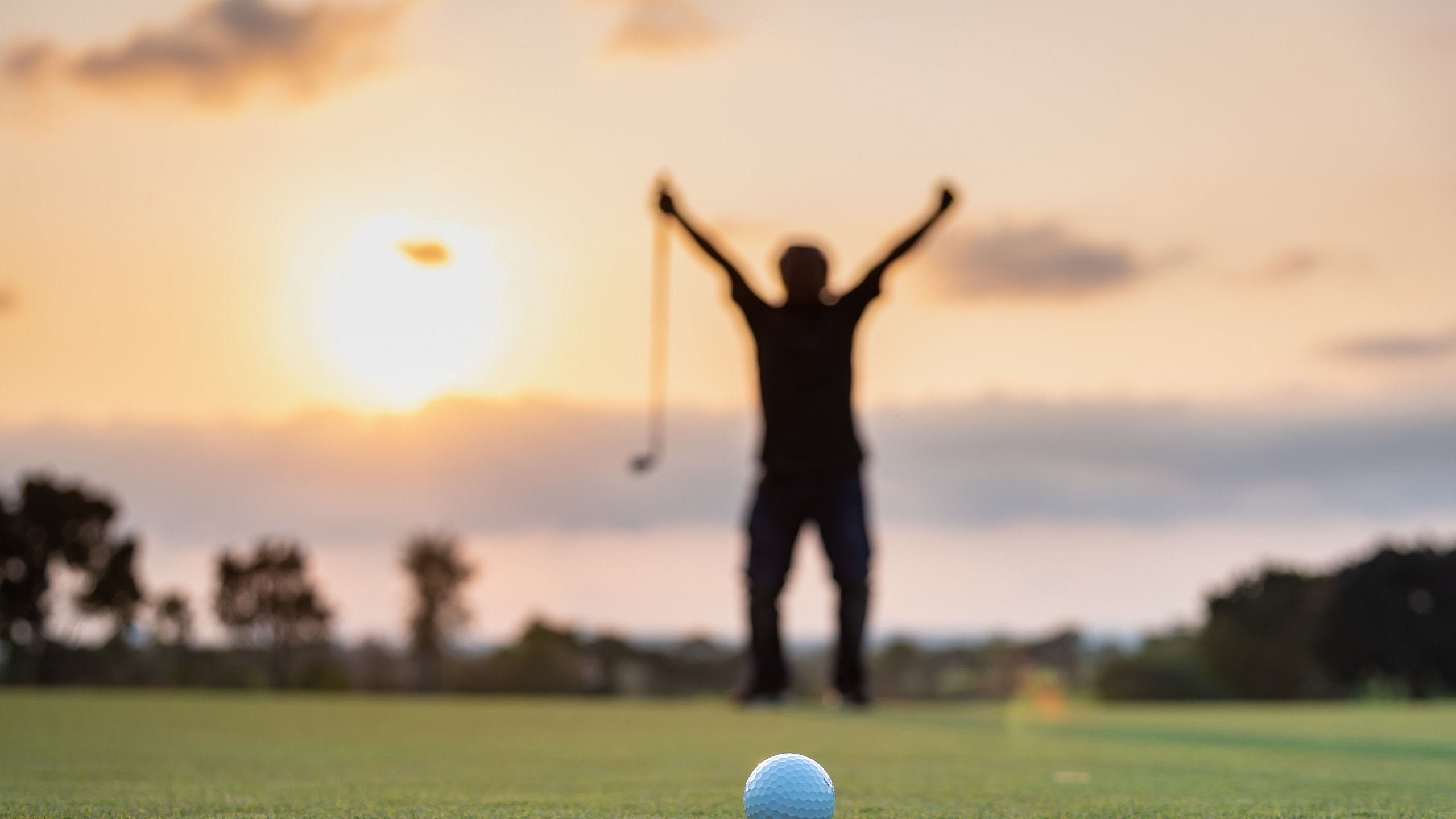In this photograph, the scene is set on a tropical golf course during sunset, characterized by a pink and purple sky, possibly Florida. The foreground is in sharp focus, capturing the intricate details of a white golf ball with indentations, positioned on the green grass at the bottom center of the image. The background is notably blurry, creating a dreamy, out-of-focus effect that only hints at the elements behind. These include fuzzy outlines of palm trees and other vegetation. Central to the image, a silhouetted male figure stands with both arms raised in a V for victory pose, holding a golf club in one hand, suggesting a celebratory moment, despite the ball not being in a hole. Mid-air is a small black dot, potentially a bird or a helicopter, adding to the sky's picturesque quality.